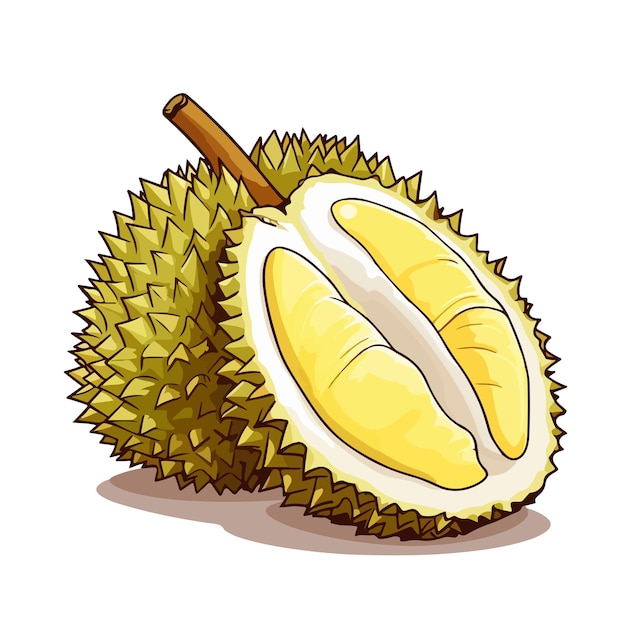The image is a detailed cartoon drawing of a durian fruit, easily distinguishable by its round, olive-green, spiky exterior. The drawing uses a palette that includes yellow, white, off-white, olive green, and brown, and features both a whole durian and one cut open to reveal the inside. The whole durian is topped with a central black stem. The cut-open durian showcases its creamy, tubular, yellow edible flesh surrounded by a white, pulpy interior layer. The depiction is not hyper-realistic but successfully represents the distinct characteristics of a durian. Notably, there is no text within the image, and it features a white background with a subtle shadow cast by the drawn fruit. The artistic rendering captures the essence of the durian, making it immediately recognizable to those familiar with the fruit.